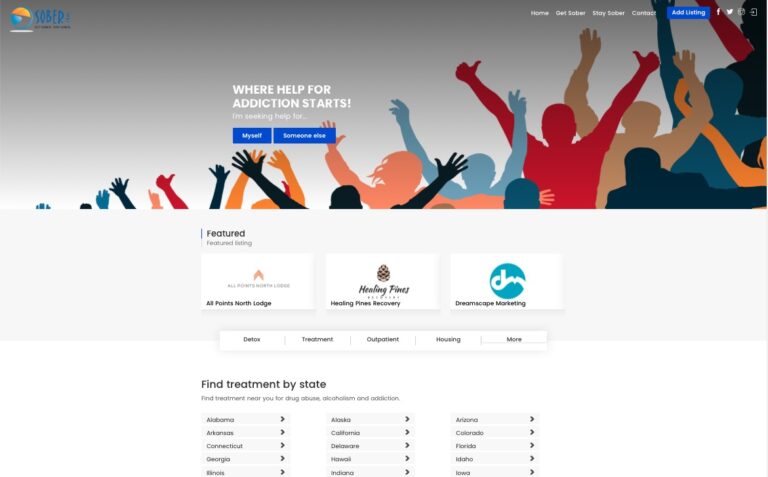The image showcases a website interface for Sober, as indicated by the logo in the upper left corner. The main graphical element includes a vibrant icon featuring silhouetted figures with raised hands, symbolizing unity and hope. These silhouettes come in various colors: teal, peach, light blue, slate gray, beige, red, and black, set against a gradient background transitioning from gray at the top to white at the bottom, reminiscent of a concert scene.

Prominently displayed in the center of the image, white text reads "Where Help for Addiction Starts!" Below this, a call to action states, "I'm looking for help... myself or someone else," with two visible blue buttons for navigation. Additional navigational options are available in the form of buttons with text such as "Home," "Get Sober," "Stay Sober," and "Curious," although they are somewhat hard to read.

On the upper right side, various icons and an ad listing are present. The central section beneath the header highlights a "Featured" area with listings for All Points North Lodge, Healing Pines Recovery, and Dreamscape Marketing, each accompanied by their logos. 

Further down, the categories include "Detox Treatment," "Outpatient Housing," and more, followed by an option to "Find Treatment by State" for drug abuse, alcoholism, and addiction. States are listed alphabetically in five rows and three columns, though the listing only covers states up to Iowa.